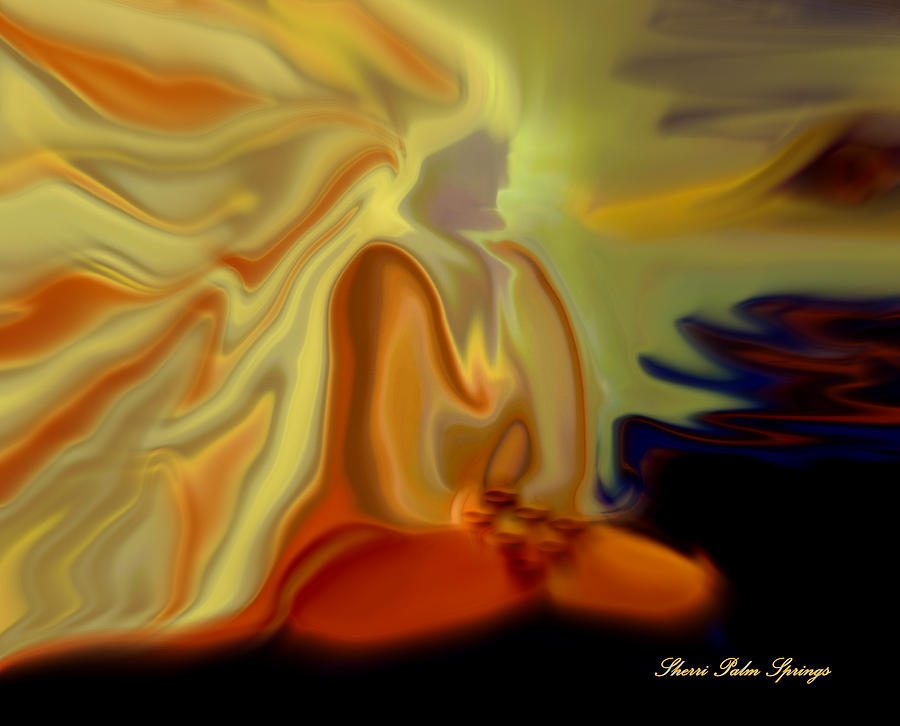This vibrant and captivating artwork, titled "Sherry Palm Springs" as indicated by the cursive yellow text in the bottom right corner, depicts a seated figure, possibly a monk or a woman, in a cross-legged, meditative pose. The person is dressed predominantly in orange, with a flowing yellowish-white top, though one description suggests a red dress. They appear to be holding something ambiguous in their hand or lap, with seven small circles adding a sense of mystery. Surrounding the central figure is an explosion of colors and dynamic lines that resemble radiant, electrifying hair cascading backward, blending shades of yellow, white, orange, red, and even some blue. The background includes purple, black, and sky-like elements, enhancing the ethereal and surreal quality of the piece. The image, which could be either a traditional painting or a digital creation, achieves a stunning contrast with the serene, central figure enveloped in a whirlwind of color and light, evoking a sense of spirituality and energy.